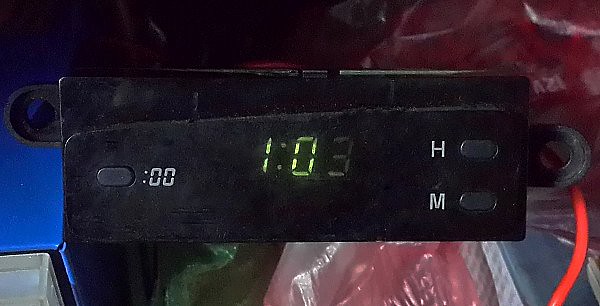This close-up photograph captures a digital clock or timer unit, likely intended for a vehicle or another electronic device due to its mounting brackets and screw tabs on either side. The black casing houses a digital display, which currently shows "1:03" in fluorescent green, though the "3" is noticeably faded. To the left of the display, there's an oval button labeled "00," perhaps for resetting the timer. On the right, two additional oval buttons are labeled "H" and "M" in white, presumably for setting the hours and minutes. A red wire protrudes from the right side of the unit, indicating a connection point for wiring. Surrounding the clock, various objects can be seen, including a dark blue toolbox with clear drawers on the left and some red plastic materials on the right. The unit is positioned on what appears to be plastic bags.